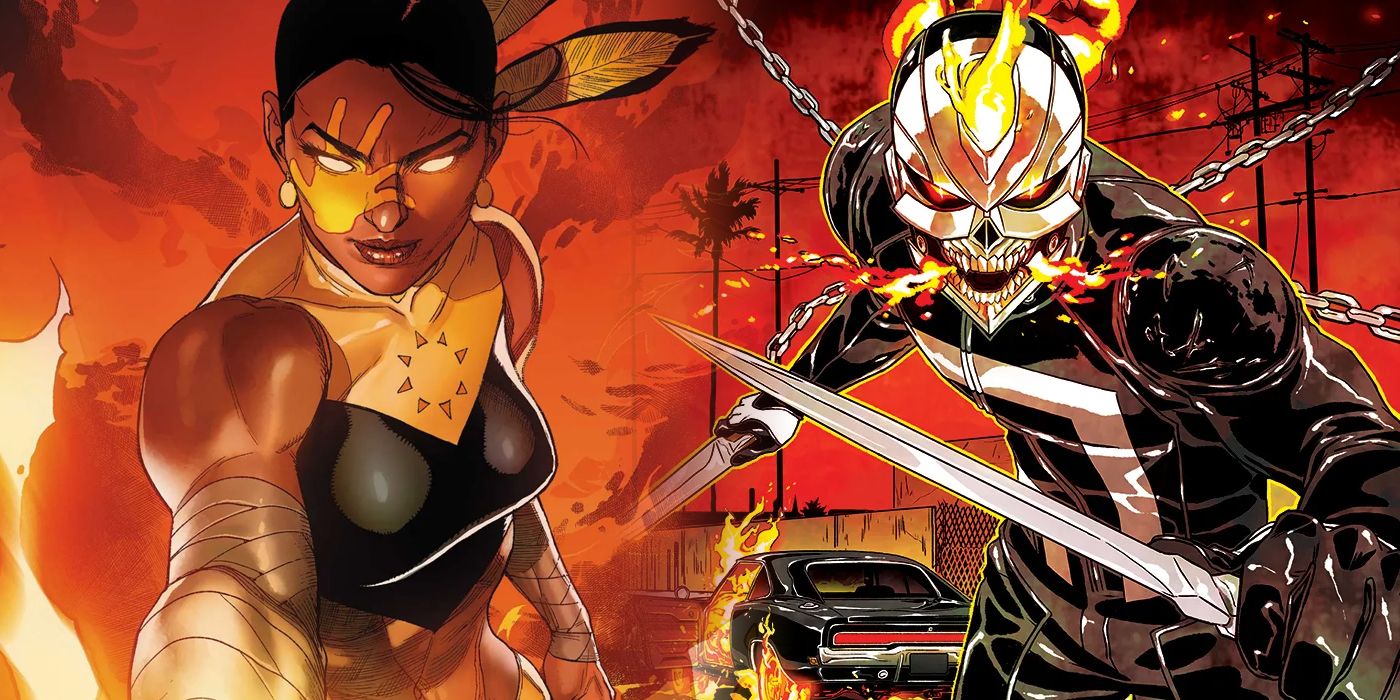The graphic image features an intense fiery red background depicting a cityscape engulfed in flames, with power lines and a possibly black car, akin to a Dodge Charger, visible in the backdrop. Center-stage are two vividly illustrated comic book characters, poised dramatically.

On the left stands Echo, the Native American deaf superhero. Echo is portrayed with a dark complexion, distinct black hair with feathers accentuating her head, and a striking yellow handprint across the left side of her face. Her glowing eyes add an intense aura to her presence. She dons a black and yellow top with triangular patterns on her chest, and her arms are wrapped in white tape around the wrist, forearm, and biceps, giving her a warrior-like appearance.

On the right is Ghost Rider, depicted as a skeletal figure with a flaming skull. He is clad in a black leather suit accentuated with metallic elements. Chains extend menacingly from his back, and he wields two daggers, engulfed in flames. Flames also emanate fiercely from his skull, enhancing his fearsome look. The scene is dynamic and full of energy, characteristic of comic book artistry, spotlighting the dichotomy between the characters' appearances and powers amidst a chaotic, fiery backdrop.